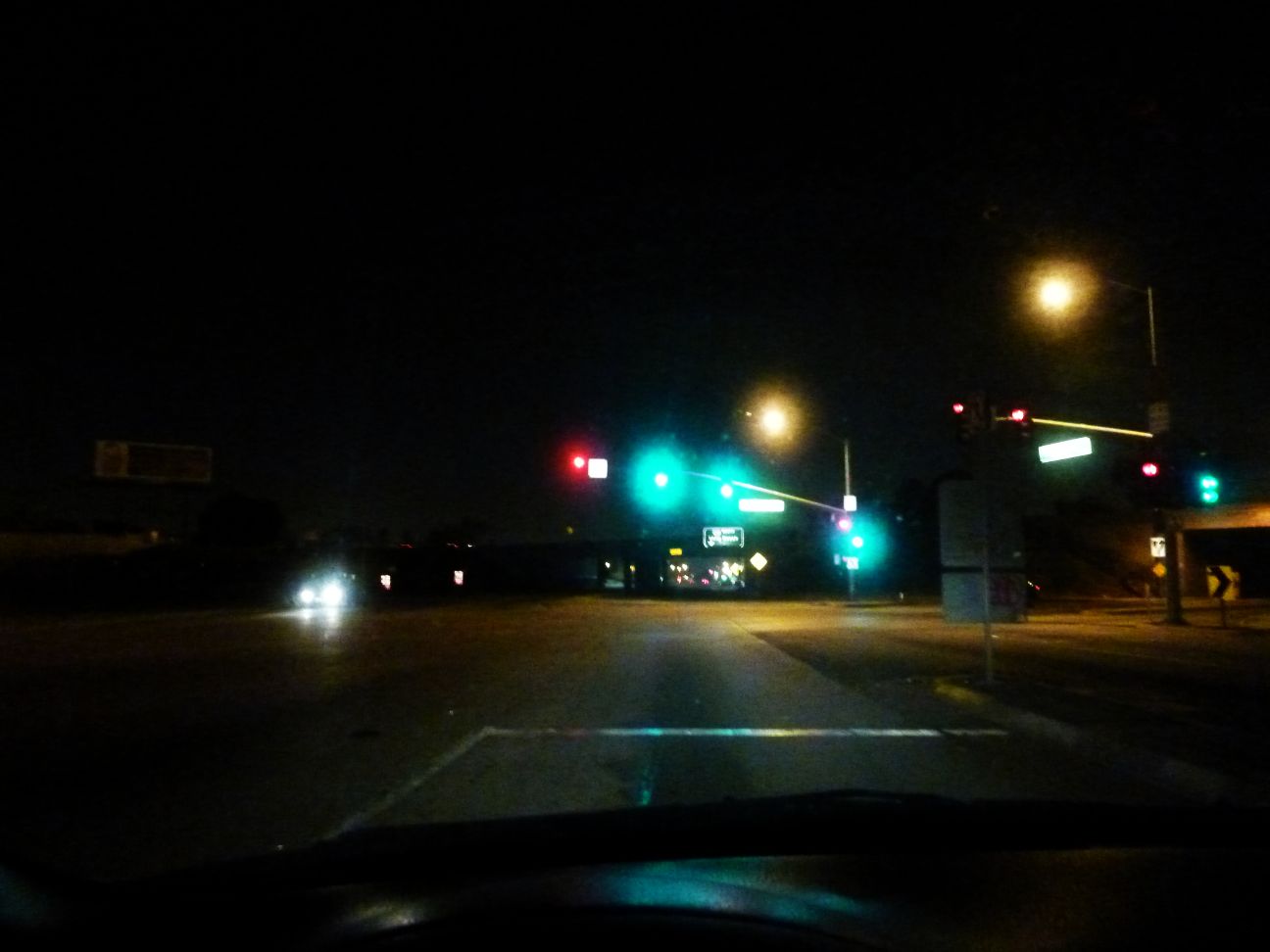Captured from inside a dimly-lit car, this evocative evening scene depicts a dark street under a pitch-black sky. The car's hood is faintly visible in the foreground, emphasizing the viewer's perspective from within the vehicle. On the right side of the street, two streetlamps cast their blurry, yellowish light, punctuating the enveloping darkness. In the distance, the soft glow of a green traffic signal adds a touch of color to the nocturnal tableau. To the left, an approaching car's bright headlights create a vivid glare, slicing through the obscurity. Far ahead, an overhead highway sign looms subtly, guiding drivers towards their destinations. Faint, blurry lights further along the street suggest the presence of distant stores or additional streetlights, barely piercing the night's thickness. This image encapsulates the stillness and subtle intrigue of a nighttime drive.